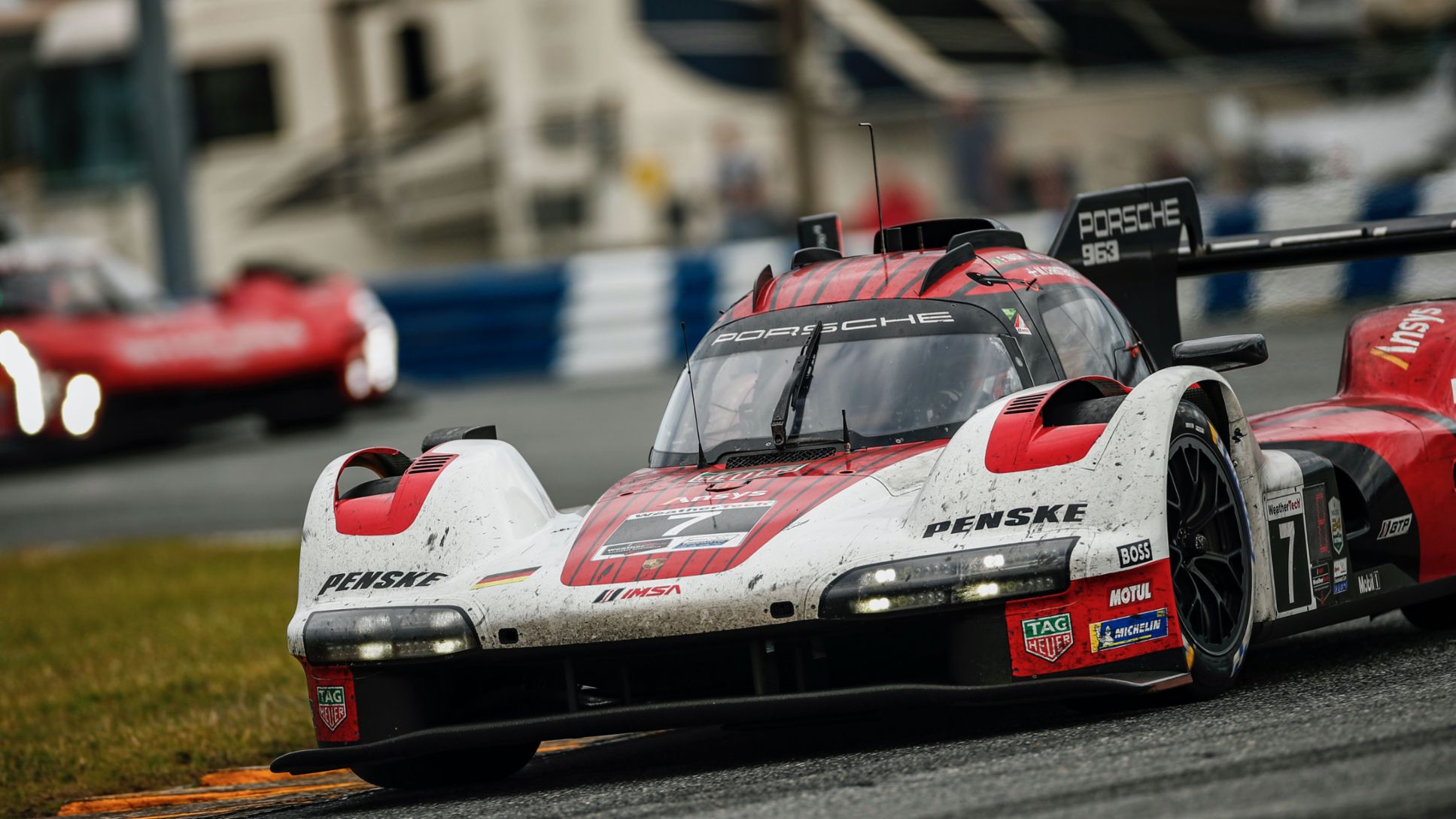The image showcases a vibrant scene on a racetrack, featuring two racing cars. Dominating the center foreground is a dynamic Formula One car, primarily white with striking red and black accents. This Porsche-branded vehicle, adorned with logos from sponsors such as Porsche, Penske Oil, Mobil Oil, Tag Heuer, and Michelin, cuts an aggressive figure with tinted windows concealing its interior, a vertical windshield wiper, wheel covers, and a small antenna atop. The distinct number 7 is visible on its body, along with bold red and black stripes and details near the headlights.

To the right, a blurred red car trails behind, emphasizing the sense of motion and competition. The asphalt track beneath them is a dark charcoal gray, bordered on the left by a vivid patch of green grass. In the distant background, you can make out a blue and white barrier and blurry figures behind, adding to the lively atmosphere of the race.